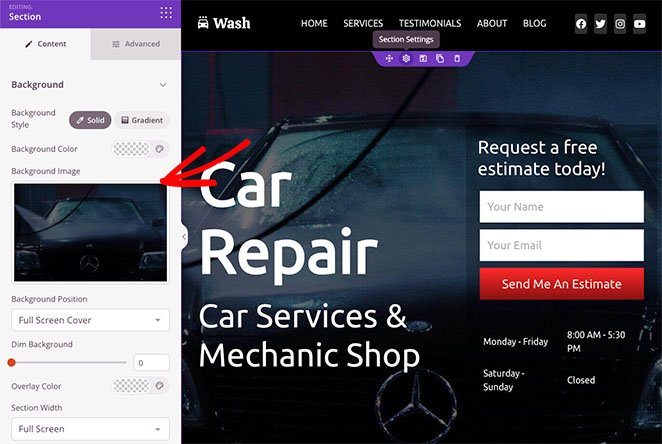The image displays a vibrant and colorful web page with a dual-frame layout. On the vertical left frame, set against a white background, a purple bar at the top bears the word "Section" in white text. Below the bar, the word "Background" appears in dark gray, accompanied by additional gray text and a faint, grayed-out image of a car. A prominent red arrow points leftward toward this dimmed image. The larger right-hand portion of the screen prominently features a brightly colored car image. Beneath the red arrow, the text "Car Repair, Car Services, and Mechanic Shop" is written in white. Further down, towards the middle right side of the image, smaller white text reads "Request a free estimate today." Directly below this text, there are two white text boxes and a red button labeled "Send Me an Estimate."